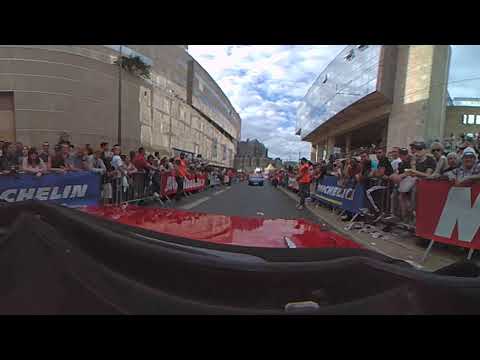This image is a daytime, outdoor color photograph taken from what appears to be a dash cam or possibly the driver’s front passenger seat of a bright red vehicle participating in an auto race. We are looking out through the windshield, flanked by black bars at the top and bottom, suggesting it is a still from a video. Ahead of us lies a gray road lined with metal barricades that keep large crowds of spectators at bay. These spectators, dressed in various colorful outfits, are on both the left and right sides, standing in front of tall buildings. Two men in orange safety vests are stationed beside the road, one on the left and one on the right. There are banners with advertisements, including notable blue Michelin signs and other red and white banners. A gray vehicle is visible in the distance ahead on the road. Above, the partly cloudy sky shows hints of blue peeking through fluffy white clouds.